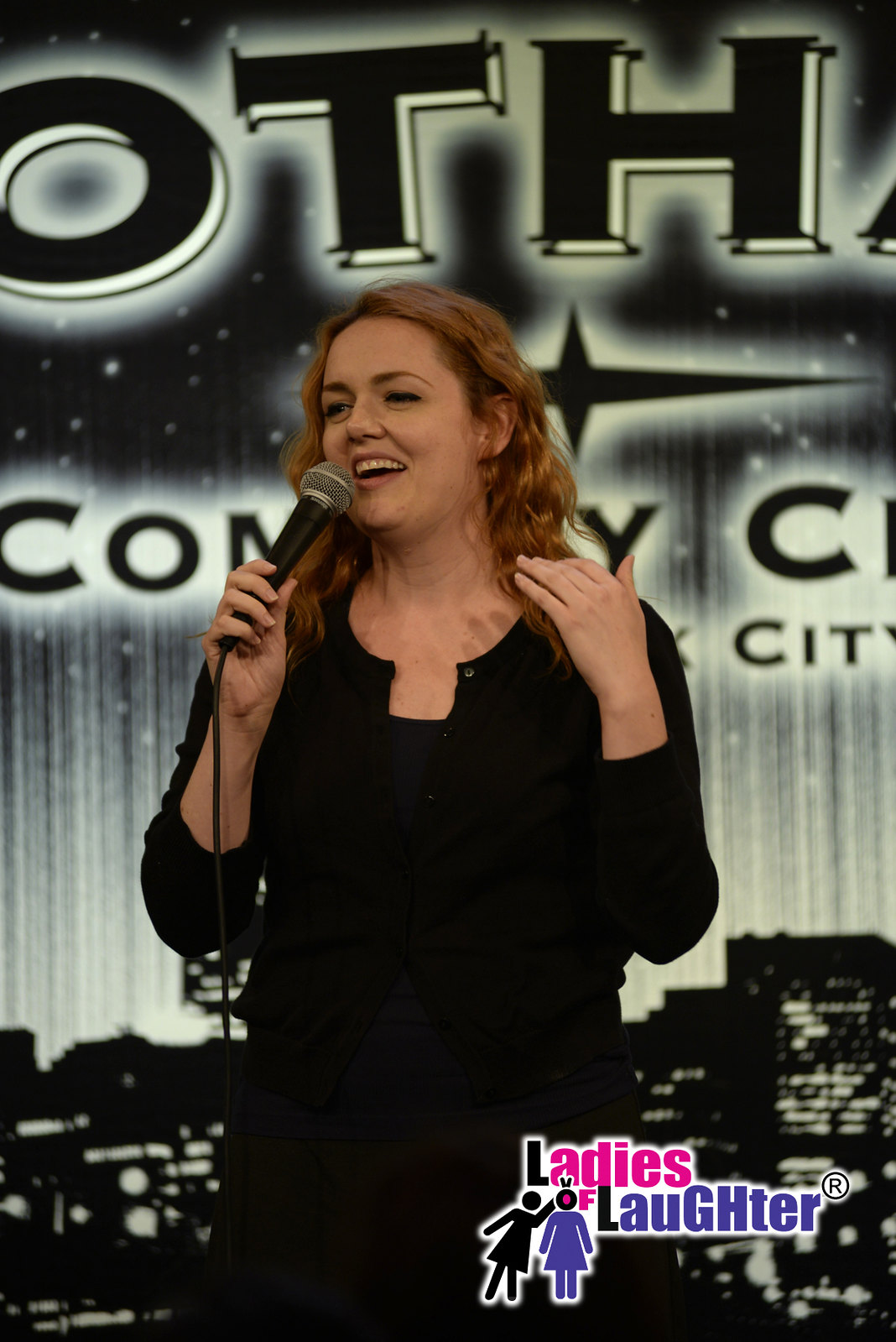The color photograph captures a woman on stage delivering a speech or performance. She is standing centered in the image, visible from the waist up, dressed in a black outfit comprising black pants, an unbuttoned black sweater, and a black top underneath. The woman, who has reddish-brown hair, holds a black microphone in her right hand; the microphone features a flexible black wire and a silver grill pointing towards her partially open mouth, revealing the top row of her teeth. She appears to be smiling slightly and gesturing with her left hand. The backdrop behind her resembles a night sky transitioning into a city skyline with lit skyscrapers. Partially visible black lettering with a white drop shadow reads "OTH" at the top and "COMEDY CITY" towards the middle, though the text is partially cut off. In the bottom right corner of the image is a watermark logo for "Ladies of Laughter," featuring two stick-figure women in dresses, one playfully giving the other bunny ears. This detailed scene embodies a dynamic and engaging moment, capturing the essence of comedic performance.